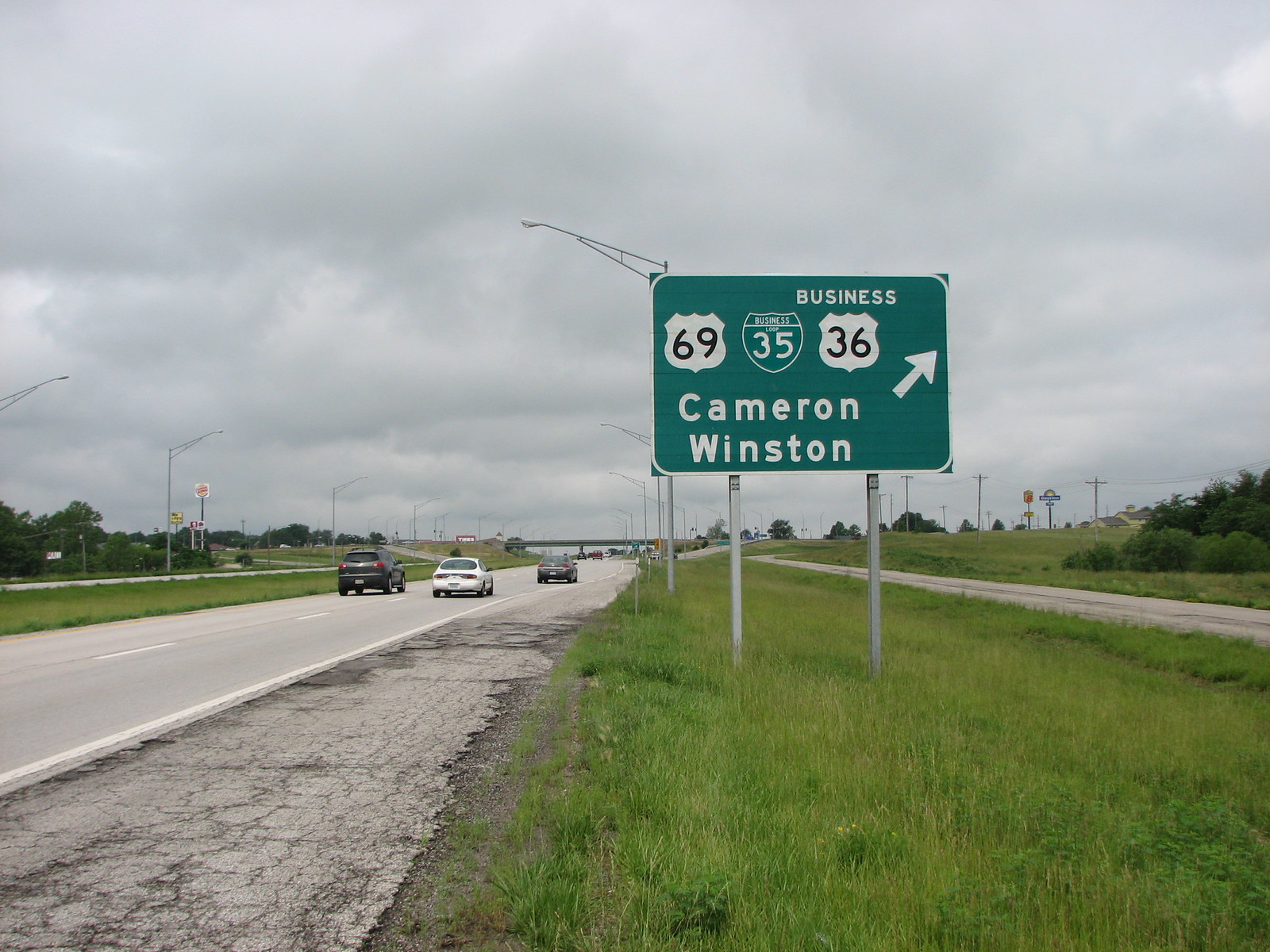The image captures a horizontal, daytime scene of a highway under an overcast sky, with green grass lining the sides. On the left side of the image is a tar road marked with white lines, featuring cars—including a black car, a white car, and a grey car—driving away towards a grey bridge situated centrally in the distance. 

Dominating the right side of the image stands a large, rectangular, green street sign mounted on two green poles. The sign features several key details: "Business" is written at the top, with an arrow pointing to the top right (northeast). Below it, on the left, is the highway number 69 in black against a white background; in the center is Business 35 in white against a green background, outlined in white; and adjacent to it is 36 in black against a white background. Below these numbers is the text "Cameron-Winston" in white lettering. 

Additional street signs are visible on both the left and right sides of the image, contributing to the sense of an intricate road network. The overall atmosphere is one of a busy, potentially worn highway stretching into the distance, under a cloudy, expansive sky.